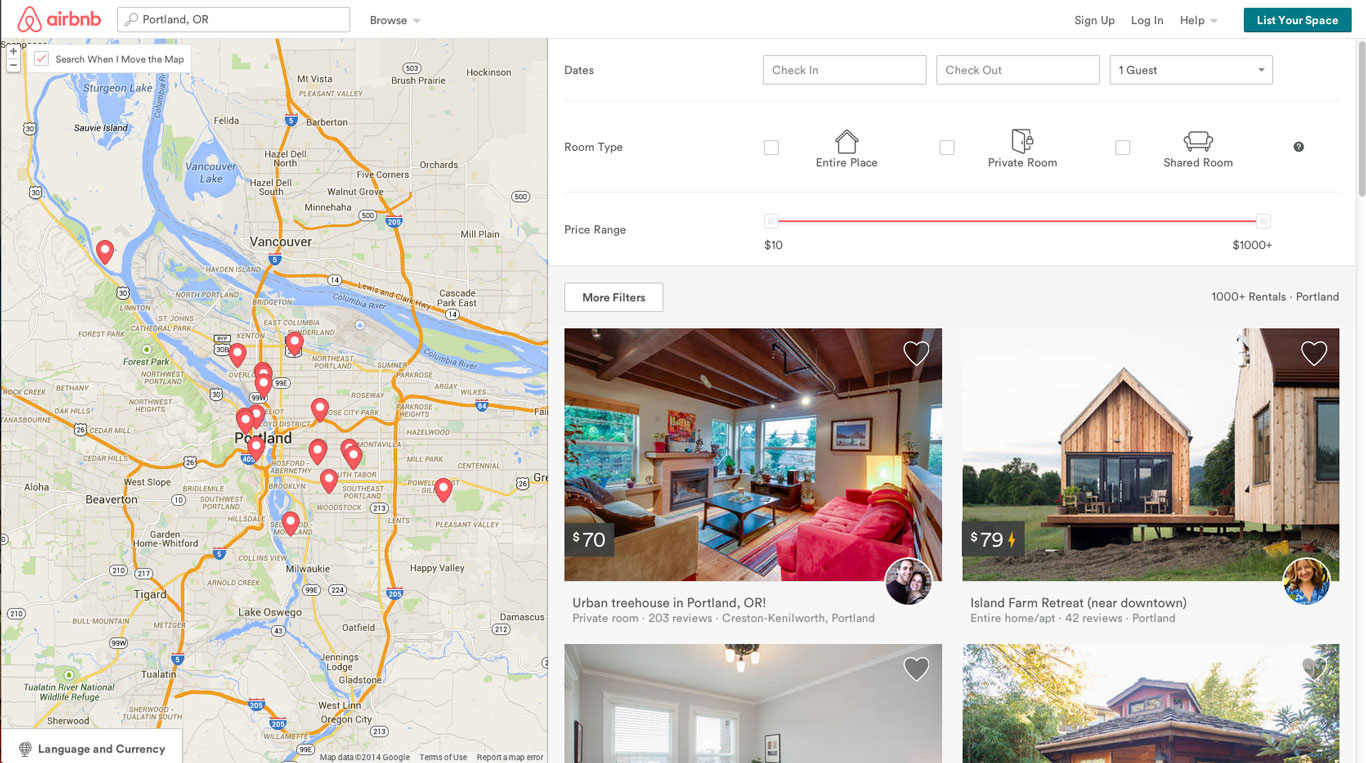This image shows a search results page for Airbnb listings in Portland, Oregon. The left side of the screen displays a map with 15 red dots representing available Airbnb locations, which extend up to include parts of Vancouver. The right side of the screen features a vertical list of Airbnb listings, each accompanied by descriptions and prices. At the top of the right panel, there are filters for selecting dates with check-in and checkout input boxes, as well as a guest drop-down menu. Below this, options to choose the type of room—entire place, private room, or shared room—are available. Additionally, a price range slider bar is positioned at the bottom, allowing users to set their budget between $10 and $1,000 or more.